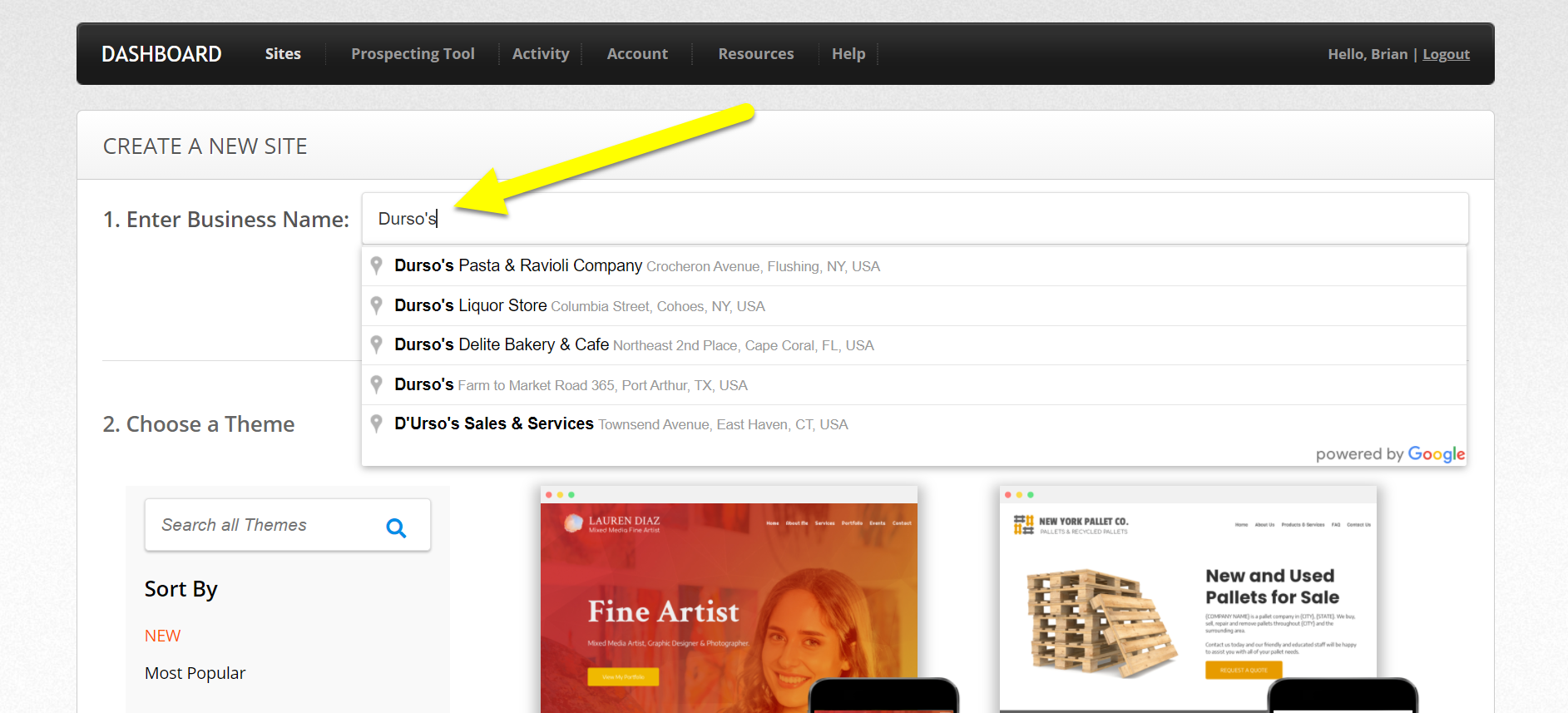This image is a screenshot of a web application interface, featuring a prominent black header. On the top left of the header is a label indicating the current section, "Dashboard." To its immediate right, a series of tabs are listed in the following order: "Sites," "Prospecting Tools," "Activities," "Account Resources," and "Help." On the far right of the header, a "Logout" link and a personalized profile link labeled "Hello Brian" are present.

In the main content area of the webpage, there is a highlighted box titled "Create a New Site." This section is divided into two rows. The first row prompts the user to "Enter a Business Name," with a yellow arrow pointing specifically to this text input field. Entering a business name, such as "Durso's," triggers a pop-up below the text bar offering suggestions for spelling or clarifying which "Durso's" the user means, along with accompanying addresses.

The second row is labeled "Choose a Theme," which includes a search box on the left side of this section. Directly beneath the search box are sorting options labeled "Sort by: New" and "Sort by: Most Popular." In the main body of the webpage, two theme options are displayed in screenshot form. The left screenshot features the title "Fine Artist," while the right screenshot showcases "New and Used Palettes for Sale."